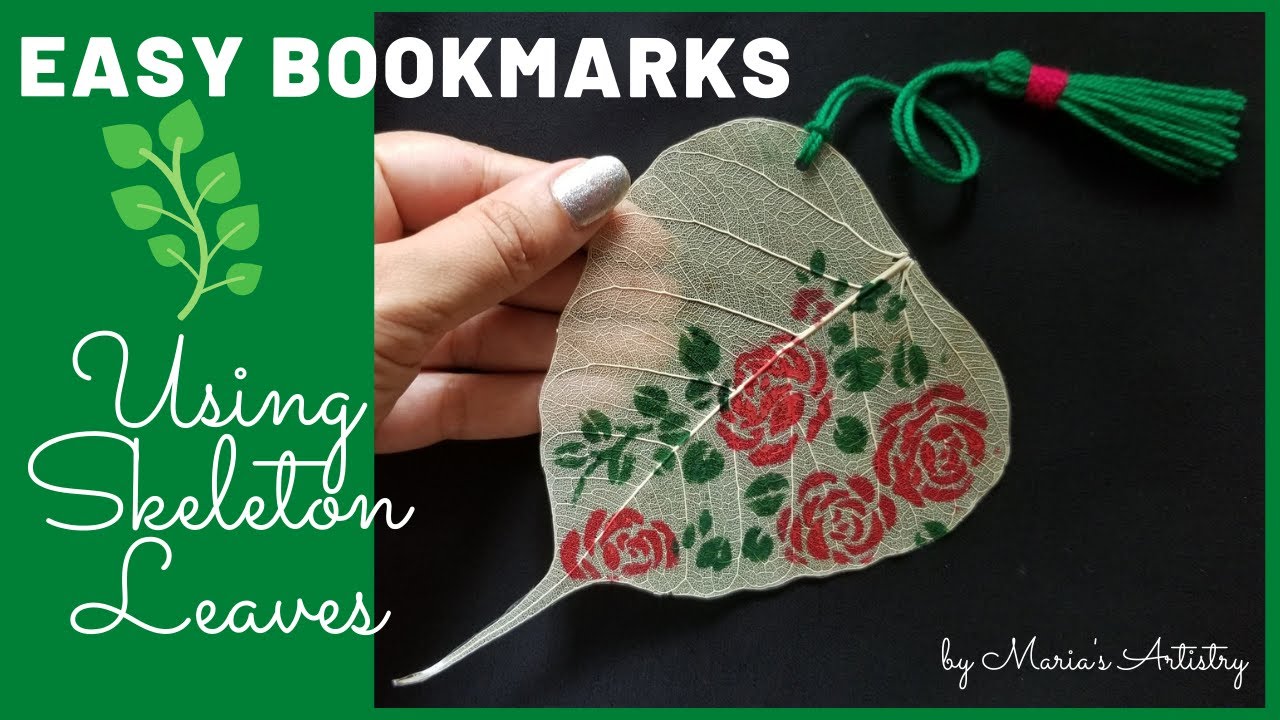The image is a landscape-oriented rectangular photograph featuring an advertisement for bookmarks. The design is split horizontally, with a green background on the left and a solid black background on the right, all bordered by a green frame. In the upper left corner, bold white block letters state "EASY BOOKMARKS," followed by an illustration of a stem with attached leaves. Below this, in white cursive letters, the caption reads "using skeleton leaves," all centered beneath each other.

Dominating the right side of the image, over the black background, is a close-up of a female hand (wearing silver glittery nail polish) holding a tear-shaped, translucent bookmark. This bookmark features a decorative red rose with green leaves painted on it. A hole punched through the top left of the bookmark holds a green tassel secured with a red tie. The hand is positioned coming from the left side, gripping the bookmark with thumb and fingertips.

In the lower right corner of the bookmark, white cursive text reads "by Maria's Artistry." The scene combines photographic realism with graphic design, merging real photographic elements with illustrative text and imagery for a visually appealing advertisement.